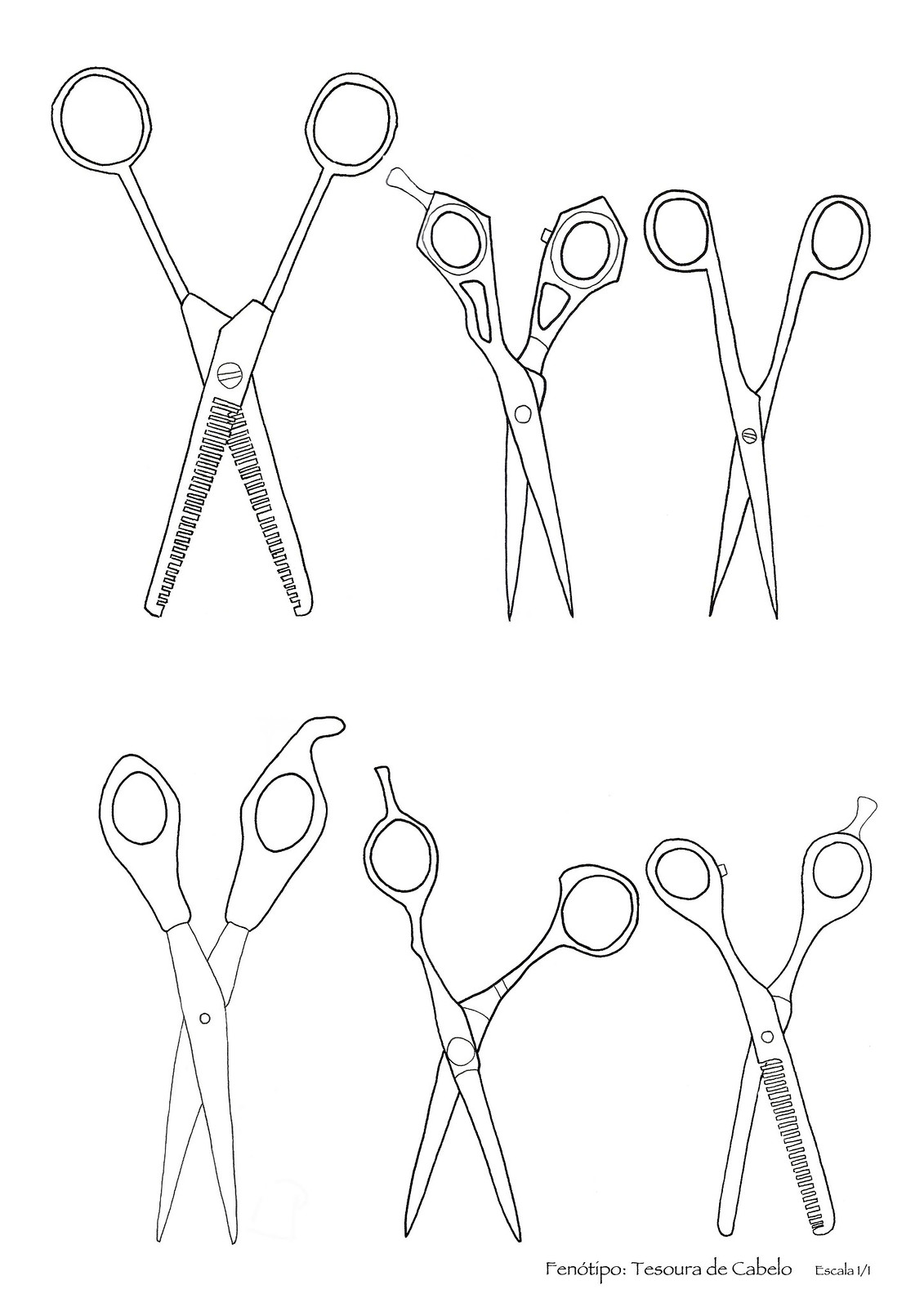This detailed pen-and-ink drawing on white paper features six distinct styles of hair scissors, meticulously arranged in two rows of three. Each scissor is crafted with unique attributes to suggest different uses in hair cutting. The scissors vary in size and blade type, highlighting the artist's attention to detail. 

In the top row, the leftmost pair of scissors features a comb-like blade, typically used for thinning hair. Next to it is a slender, long-blade pair designed for precise, sharp cuts. The rightmost in this row is a shorter, stubby pair, possibly for beard trimming, with a robust, sharp appearance.

The bottom row mirrors the arrangement, starting again with a thinning shear on the left, similar to the top left but slightly different in size. The middle and right pairs in this row are longer, sharp-bladed scissors meant for general hair trimming.

The image also contains Spanish text at the bottom in black font: “F-E-N-O with an accent, T with an accent, P-O... TESOURA DADE CABELO Escala 1/1,” which emphasizes the artistic and functional aspects of the scissors. The overall black-and-white composition underscores the utilitarian beauty of these essential hairdressing tools.